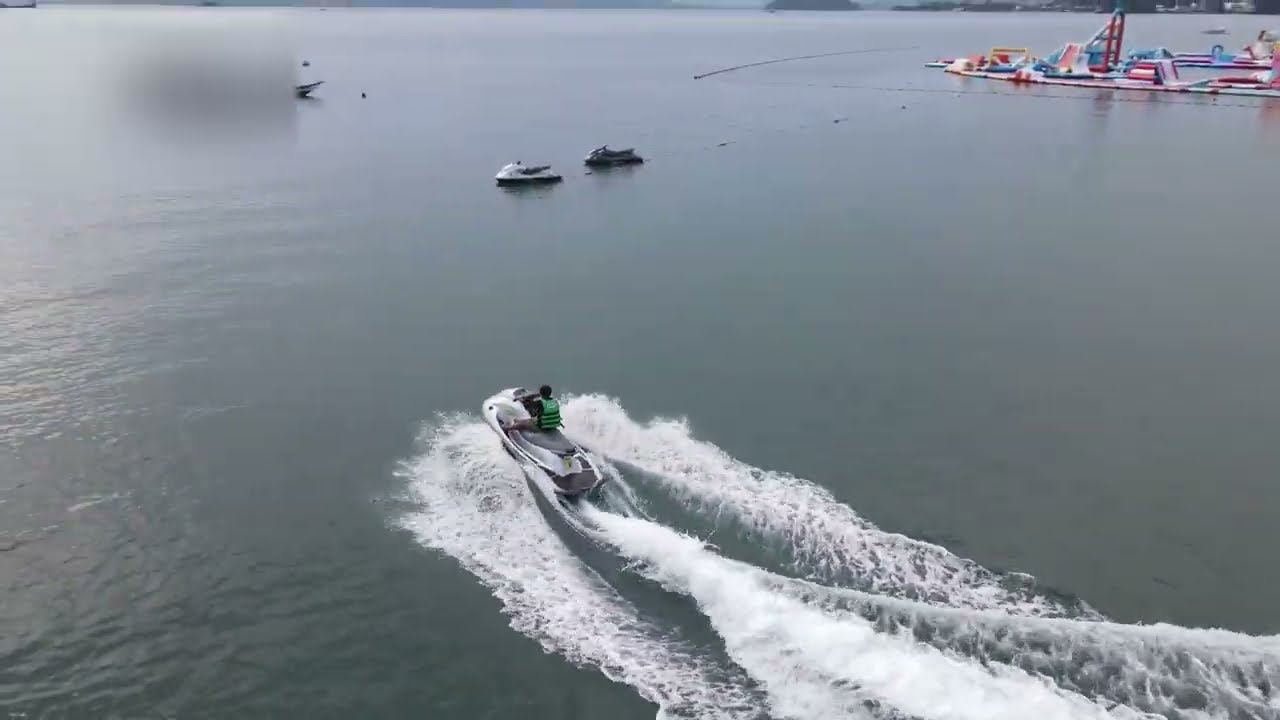The image depicts a large body of water, possibly a lake or a bay, during an overcast and dreary day. The water, which dominates the picture, is a dark blue-gray, reflecting the hazy gray sky. In the foreground, a person is speeding away from the camera on a black and white jet ski, creating a significant white wake behind him. He is wearing a green and black striped lifejacket. To his right, a white and gray jet ski floats unattended, facing left. In the lower right-hand corner is this stationary jet ski. The center of the image, slightly to the left, features a blurred-out boat or ship, obscured except for the very top of the wheelhouse. In the far distance, other boats can be seen along with large, dark gray mountains partially obscured by low clouds and fog. Some rolling hills and small islands are visible to the right, and a buoy line runs across the upper right-hand portion of the image, suggesting proximity to the shore. The overall scene is enveloped in tones of blue and gray, contributing to the gloomy atmosphere.